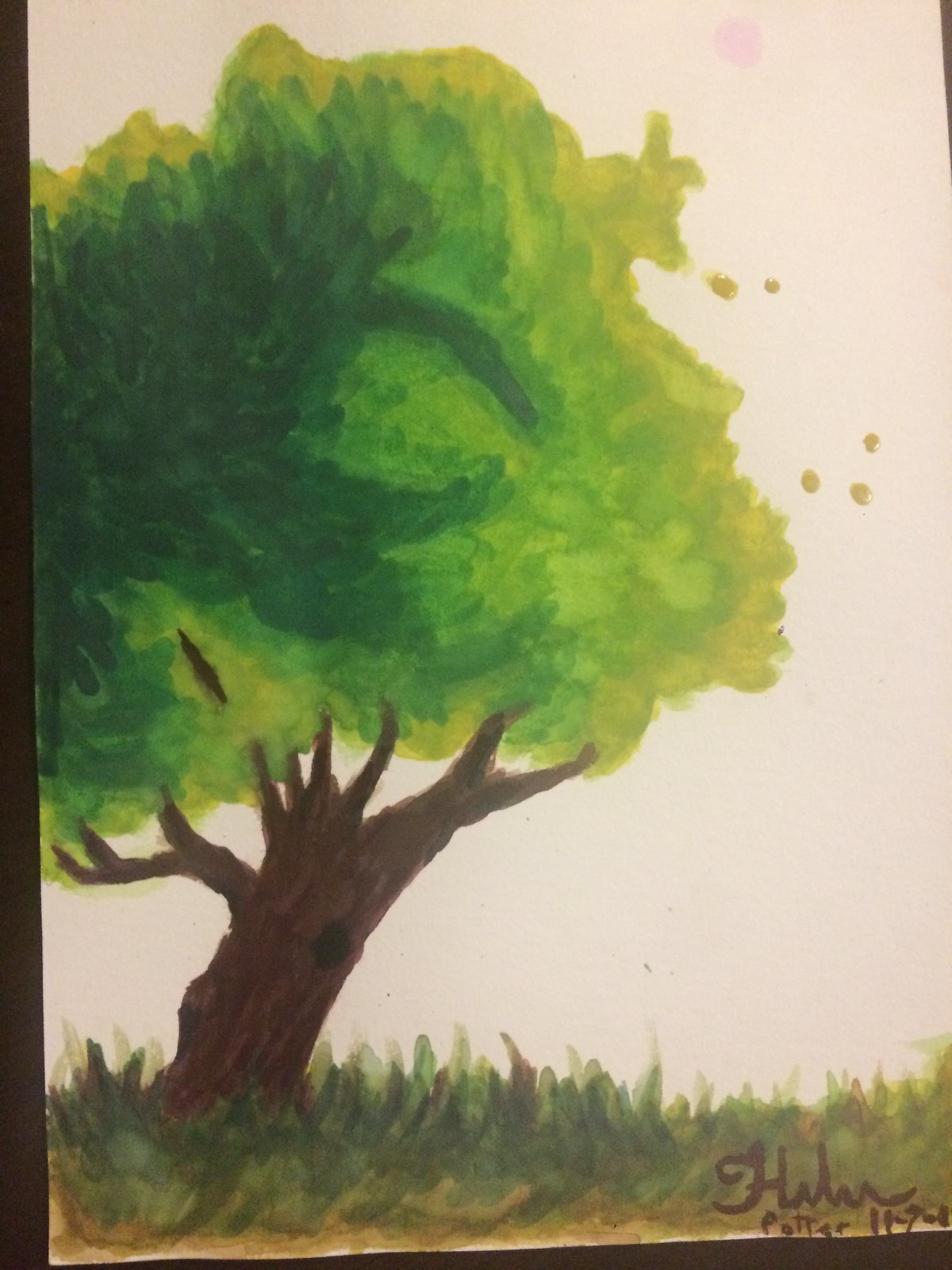A watercolor painting on white paper features a detailed depiction of a tree in a natural setting. In the top left corner, vibrant green leaves emerge, with shades transitioning from dark green on the left to light green on the right. The tree's trunk, rendered in a rich brown with black accents indicating a hollow, displays light brown marks for texture. The ground at the bottom is covered with lush green grass interspersed with patches of dry foliage in dark green and light brown hues. A prominent branch extends upwards, showcasing the artist’s skill in blending dark and light greens. In the bottom right corner, there is cursive text reading "Potter 11-...", adding a personal or possibly a signature element to the painting. The entire piece showcases a skilled use of watercolor to depict a serene and detailed natural scene.